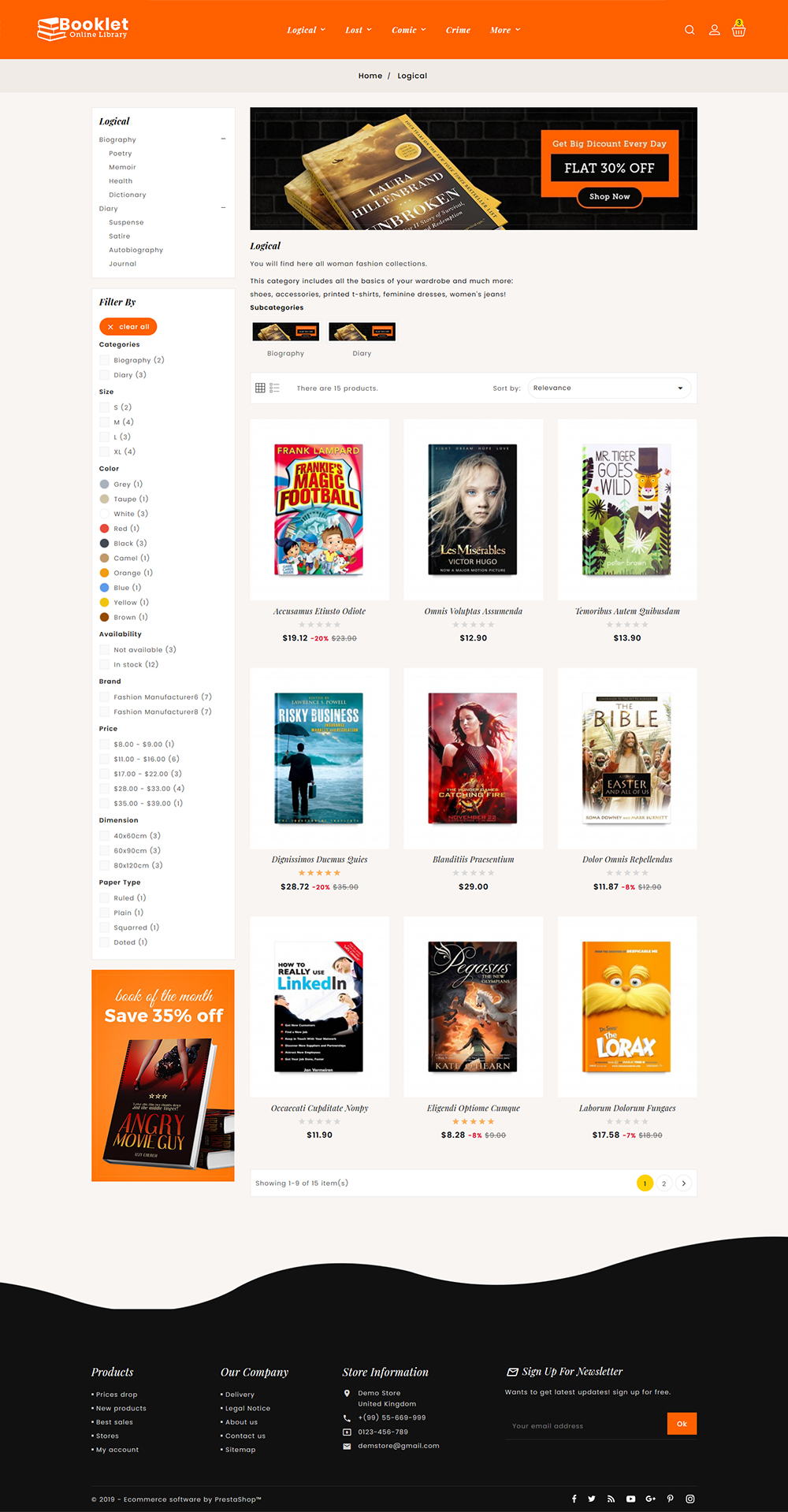The image depicts a screenshot of a digital bookstore's interface. In the upper left-hand corner, there is a heading, though its title isn't entirely clear. The top of the page features several tab options such as "Explore," along with other indistinct tabs. The upper right corner is equipped with a search icon, a profile icon, and a shopping cart icon. A prominent pop-up message offers a "Flat 30% Off" discount accompanied by a "Shop Now" button.

Below this advertisement, various book covers are displayed in a grid format. These include "Frankip's Magic Football," "Mr. Tiger Goes Wild," "Risky Business," a "Hunger Games" book, "The Bible," a book about LinkedIn, a title named "Pegasus," and "The Lorax" by Dr. Seuss. On the left side of the screen, a filter section is available, providing multiple options to refine and choose the suitable book from the collection.